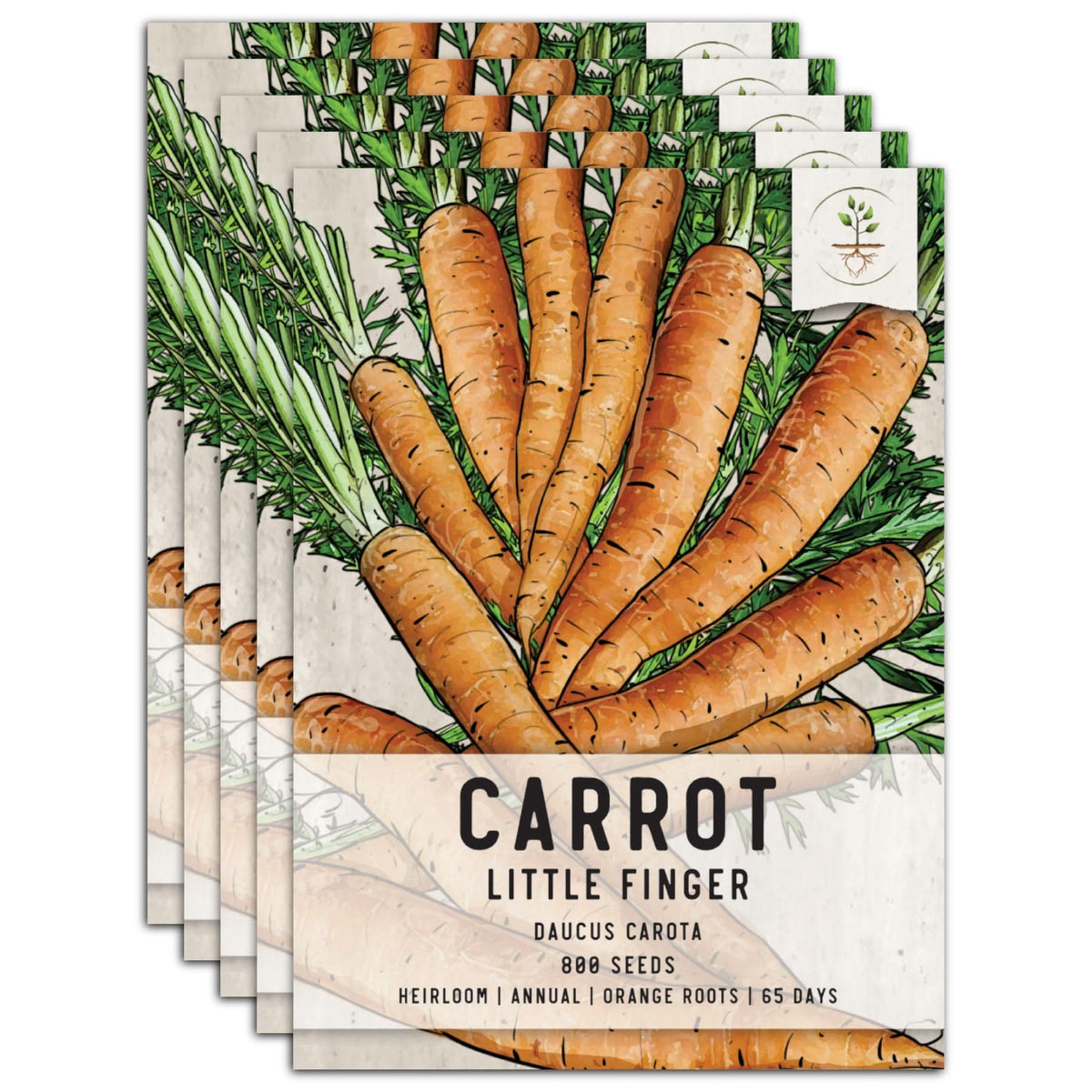This image depicts five slightly staggered, stacked bags of carrot seeds, showcasing a repeating illustration of vibrant orange carrots with green tops. Each seed packet features an intricate main image of fully grown carrots, complemented by an upper right corner drawing of a plant with visible roots, a line of earth, and five sprouting green leaves. The lower half of the packet, set against the illustrated carrots, is predominantly white and overlaid with dark text detailing the product: "Carrot, Little Finger, Daucus carota, 800 seeds, heirloom, annual, orange roots, 65 days." The carrots illustrated on the packet number eleven, vividly bunched together, emphasizing the rich, green and orange hues, indicative of the healthy produce these seeds will yield.